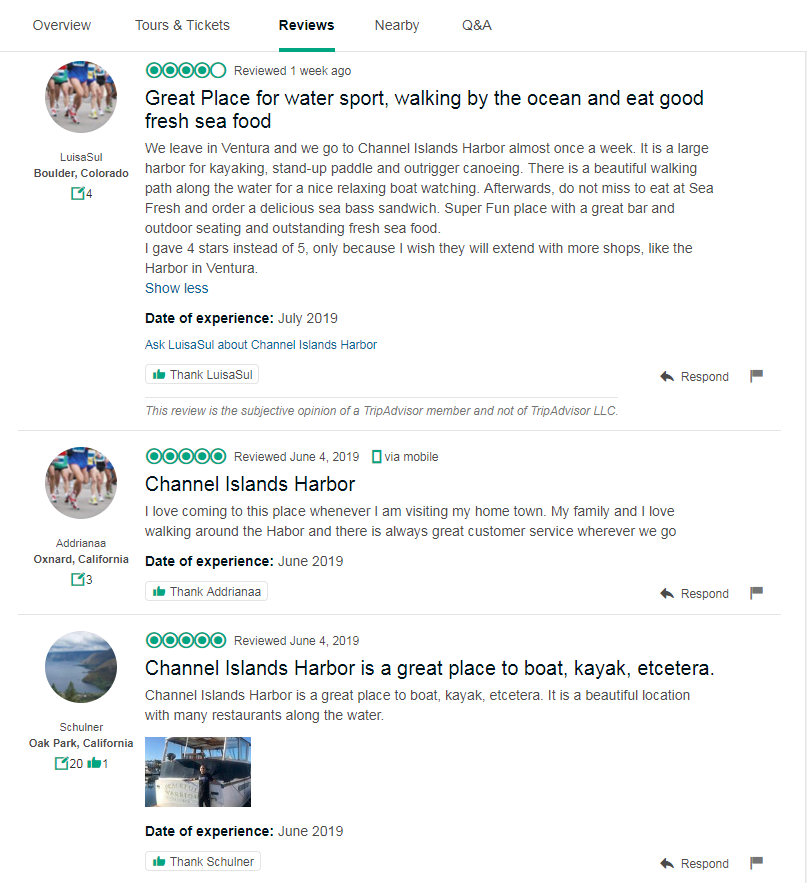**Yelp Screenshot Overview for Channel Islands Harbor, Boulder, Colorado**

At the top of the screenshot, tabs labeled *Overview*, *Tours and Tickets*, *Reviews* (selected), *Nearby*, and *Q&A* are visible, followed by a review from Louisa Soul.

---

**Review Summary:**

**Louisa Soul, Boulder, Colorado:**  
⭐⭐⭐⭐☆ (4/5 stars)  
**Reviewed: One week ago**  
**Date of Experience: July 2019**

Louisa describes Channel Islands Harbor as a "great place for water sports, walking by the ocean, and eating good fresh seafood." She lives in Ventura and visits the harbor almost weekly. The location offers a large harbor suitable for kayaking, stand-up paddleboarding, and outrigger canoeing. A scenic walking path along the water provides a relaxing spot for boat-watching. Louisa highly recommends dining at SeaFresh, especially noting the sea bass sandwich. Despite its numerous attractions and a great bar with outdoor seating, she wishes for more shops similar to those in Ventura, leading to a four-star rating.

---

**Additional Reviews:**

**Addriana, Oxnard, California:**  
⭐⭐⭐⭐⭐ (5/5 stars)  
**Reviewed: June 4th, 2019**  
**Date of Experience: June 2019**

Addriana enjoys visiting Channel Islands Harbor whenever she is in her hometown. She highlights the enjoyable walks around the harbor with her family and appreciates the excellent customer service at various venues along the waterfront.

---

**Schulner, Oak Park, California:**  
⭐⭐⭐⭐⭐ (5/5 stars)  
**Reviewed: June 4th, 2019**  
**Date of Experience: June 2019**

Schulner praises Channel Islands Harbor as a "great place to boat, kayak, etc." He mentions its beautiful location and the variety of waterfront restaurants.

---

**Summary:**

Channel Islands Harbor in Boulder, Colorado, is well-loved by visitors for its extensive water sports activities, scenic walking paths, and outstanding seafood restaurants. The harbor receives high marks for its ambiance, customer service, and dining options, although some wish for more retail development similar to nearby Ventura.